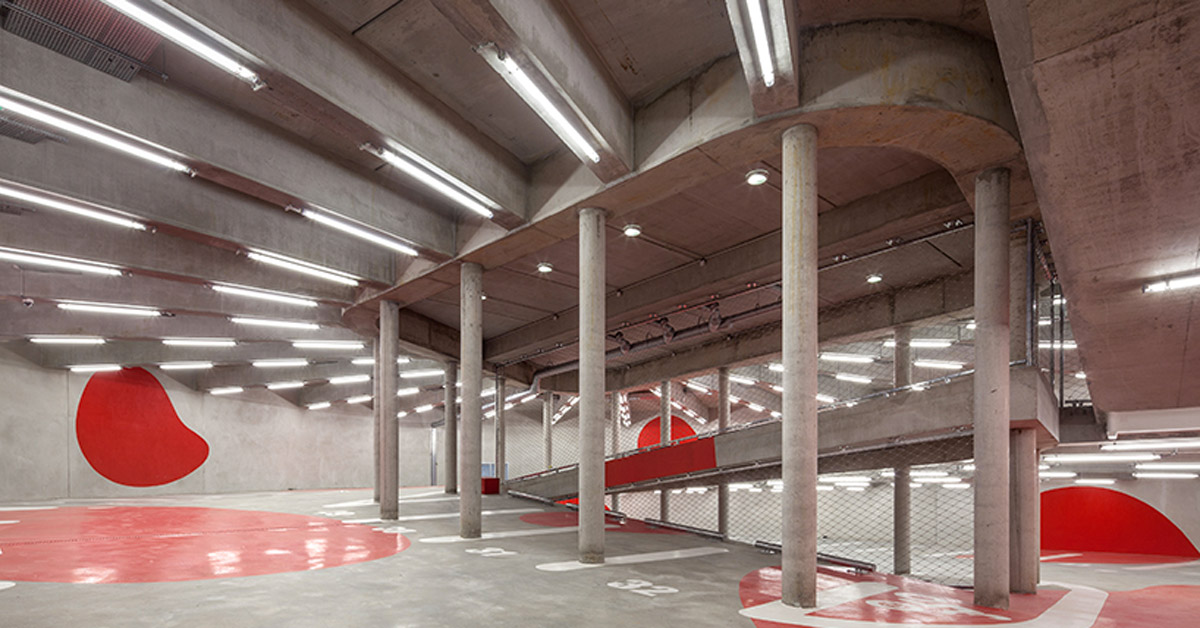This image depicts a modern, uniquely designed parking garage. The structure features a spiraling ramp that curves upward, adorned with fluorescent tube lights on every cement post across the ceiling. Red circles, which likely indicate floor levels, are painted on both the walls and the ground. The concrete floor, appearing almost mirrored, is painted silver along with the rest of the structure, enhancing its contemporary look. Distinctive steel beams and pillars support the ceiling, while the central portion of the spiral ramp has cement pillars placed periodically along its rounded edge. Each parking spot is clearly marked with white paint, displaying numbers such as 32 and 31. A notable detail includes a handicapped parking space, designated by its specific logo. In the right corner, an air vent is visible, presumably for exhaust ventilation. The color palette is predominantly silver, red, gray, and white, contributing to the sleek, modern ambiance of the parking garage.